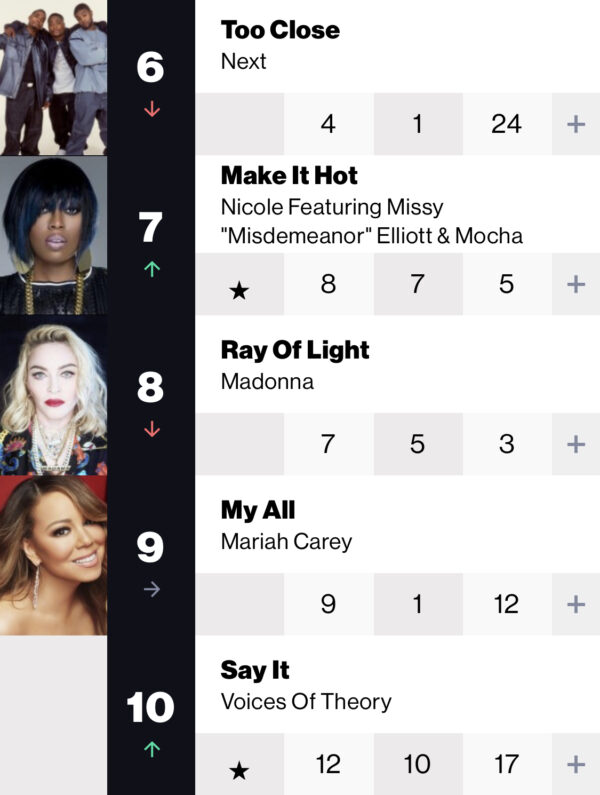**Top 10 Artists of the Week**

This rectangular screen displays this week’s top 10 artists, highlighting their positions from 6th to 10th with detailed captions. On the left side, images of the artists accompany their rankings:

6. **Boy Band Trio**: Three men are dressed in various outfits, including jean shorts, long-sleeve shirts, and pants, all fully covered. Accompanying their image is a red arrow pointing downward, indicating a drop in position.

7. **Female Artist**: A woman with short-cropped black hair wearing a golden necklace and black t-shirt. A green arrow pointing upward beside her name signifies a rise in ranking.

8. **Blonde Singer**: This artist sports shoulder-length blonde hair, a red and black jacket adorned with golden chains, red lipstick, and blue eyes. A red arrow points downward, signifying a decrease in her ranking.

9. **Brown-Haired Woman**: Featuring brown, curly hair, and dangling necklaces, her image intriguingly cuts off just above the collarbone. A purple arrow pointing horizontally indicates no change in her position.

10. **Gray Placeholder**: Without a photograph, this position is represented by a gray block. A green arrow points upward, illustrating an improvement in ranking.

On the right, the corresponding songs and featured artists are listed by position:

6. "Too Close" by Next
7. "Make it Hot" by Nicole featuring Missy "Misdemeanor" Elliott and Mocha
8. "Ray of Light" by Madonna
9. "My All" by Mariah Carey
10. "Say it" by Voices of Theory

Stars and numbers further indicate the ranking dynamics and provide a visually engaging summary of the artists' standings for the week.